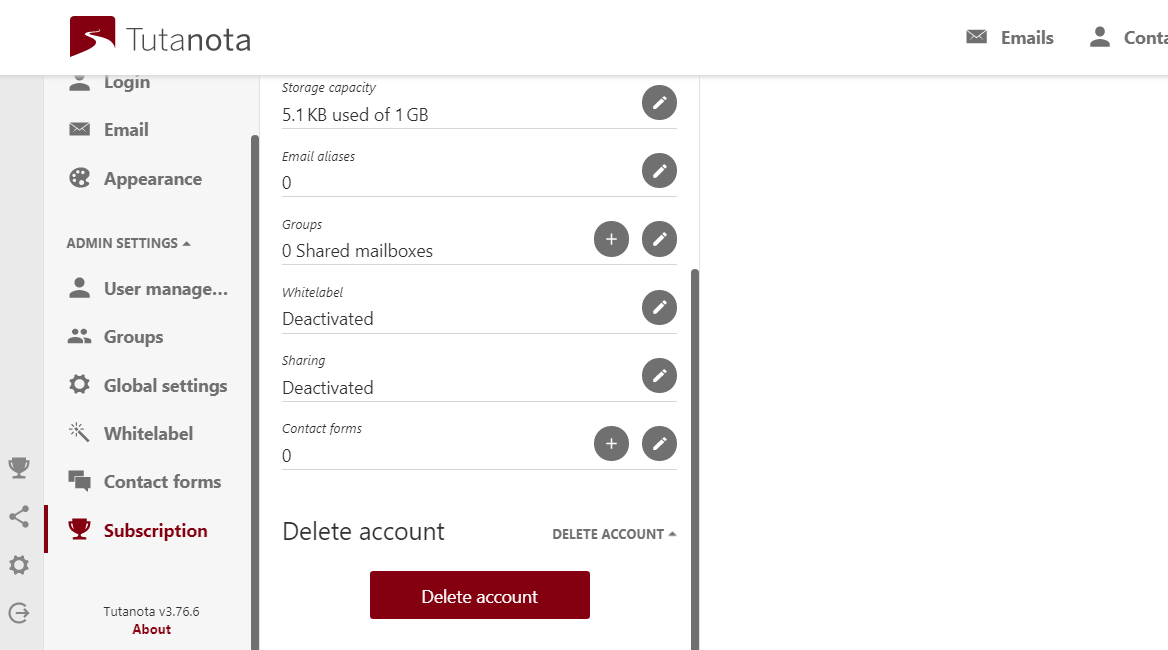The image is a horizontally rectangular screenshot featuring a primarily white background, displaying an app interface. 

At the top left corner, there's the "Tutanota" logo. To the right of the logo, partially visible, are the options for "Email" and "Contact." Some part of the right side of the app frame is cut off, causing the "Contact" option to be truncated and only showing "C-O-N-T" and a portion of the letter "A."

Based on the visible scroll bars, only a portion of the vertical options on the app interface is visible. On the left panel, the menu options include: "Login," "Email," "Appearance," "Admin Settings," "User Manage," "Groups," "Global Settings," "White Label," "Contact Forms," and "Subscription," with "Subscription" highlighted in burgundy, indicating that it is the selected option.

To the right, detailed information about the selected "Subscription" option is displayed:
- **Storage Capacity:** 5.1 KB used of 1 GB
- **Email Aliases:** 0
- **Groups:** 0
- **Shared Mailboxes:** 0
- **White Label:** Deactivated
- **Sharing:** Deactivated
- **Contact Form:** 0

In larger font, the phrase "Delete Account" is visible. Below this, centered on the screen, is a burgundy "Delete Account" button.